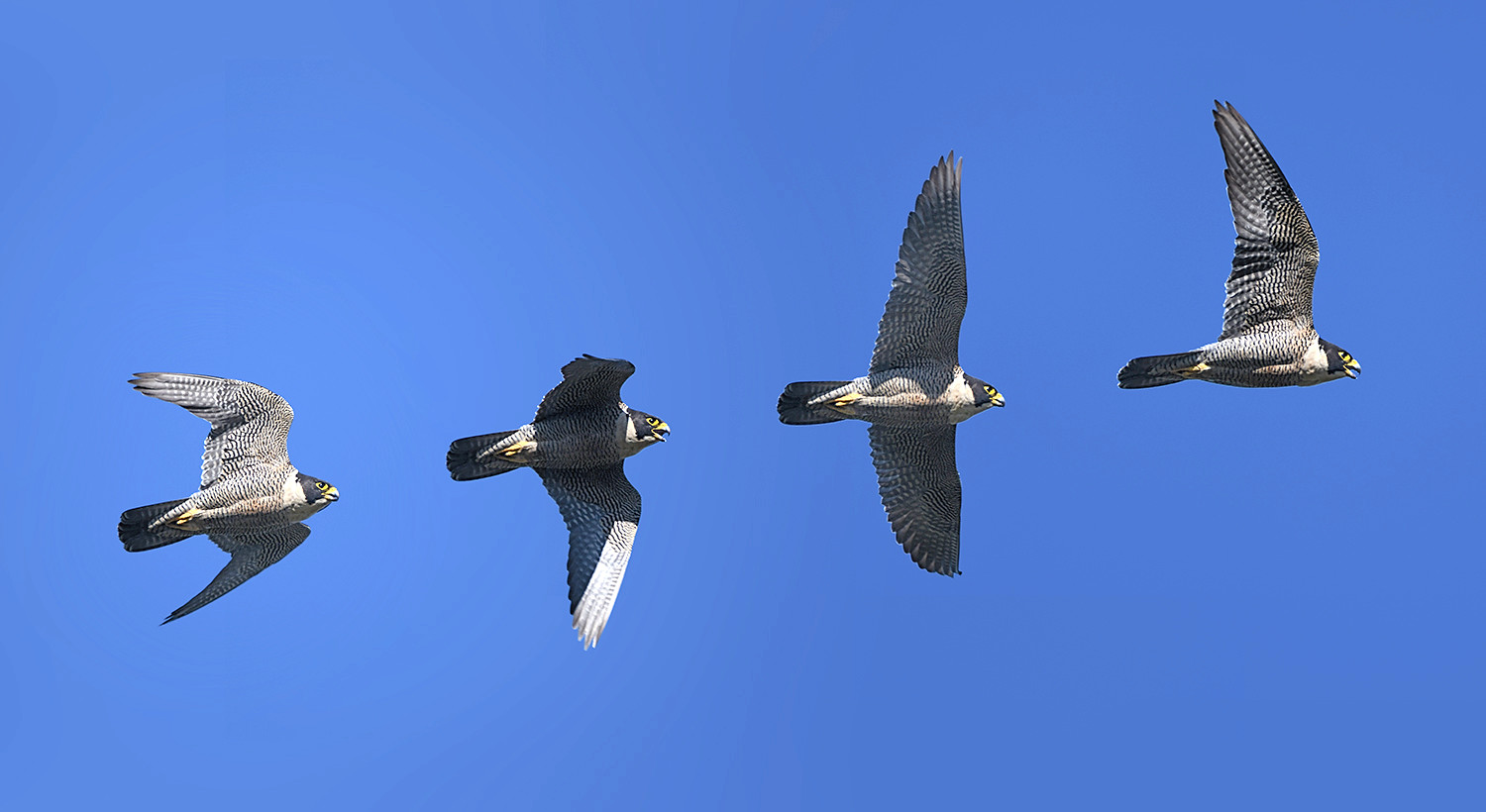A vivid daytime photograph captures a sequence of four peregrine falcons flying in a perfectly straight line from left to right against a crystal clear blue sky. The birds appear almost equidistant, creating a mesmerizing pattern as each is in a different stage of wing flap — suggesting the image might be digitally altered to show the same bird at various points in its flight cycle. The leftmost falcon has its wings in a neutral position, partially extended out. To its right, the falcon's wings are beginning the downstroke, while the third bird has its wings fully extended outward. The far-right falcon completes the sequence with its wings in the upstroke position above its body.

All four falcons display distinct features characteristic of their species: their undersides are white with dense black speckles, and they have a black triangular mask covering their eyes. Their heads are black, complemented by yellow, short, sharply hooked beaks. The birds’ tail feathers are slightly darkened with streaks of gray. The photograph is taken from a vantage point below the birds, allowing a clear view of their underside but not their topside. The remarkable image showcases both the beauty and the detailed specifics of the peregrine falcon's flight, emphasizing the sleek, powerful form of these magnificent birds in motion.